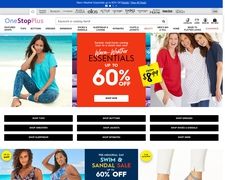Screenshot from the One Stop Plus e-commerce website:

On the far left side of the image, the One Stop Plus logo is prominently displayed with "One" in blue, "Stop" in dark purple, and "Plus" in lilac. Across the top of the website, there are approximately ten navigation tabs. Beneath these tabs, there are various promotional images. In the middle section, an orange box with white text announces a 60% off discount on essentials, accompanied by a prominent "Shop Now" button. To the left of this box, a model is seated on a beach, while on the right side, three women are smiling joyfully. The layout is clean and straightforward.

Below this section, there are nine black buttons, each representing different categories of clothing items, with the text on these buttons in white. Further down the page, another advertisement features two women standing on a beach, dressed in summer attire. In the center of this ad, white text in an orange box highlights a sandal sale offering 60% off.